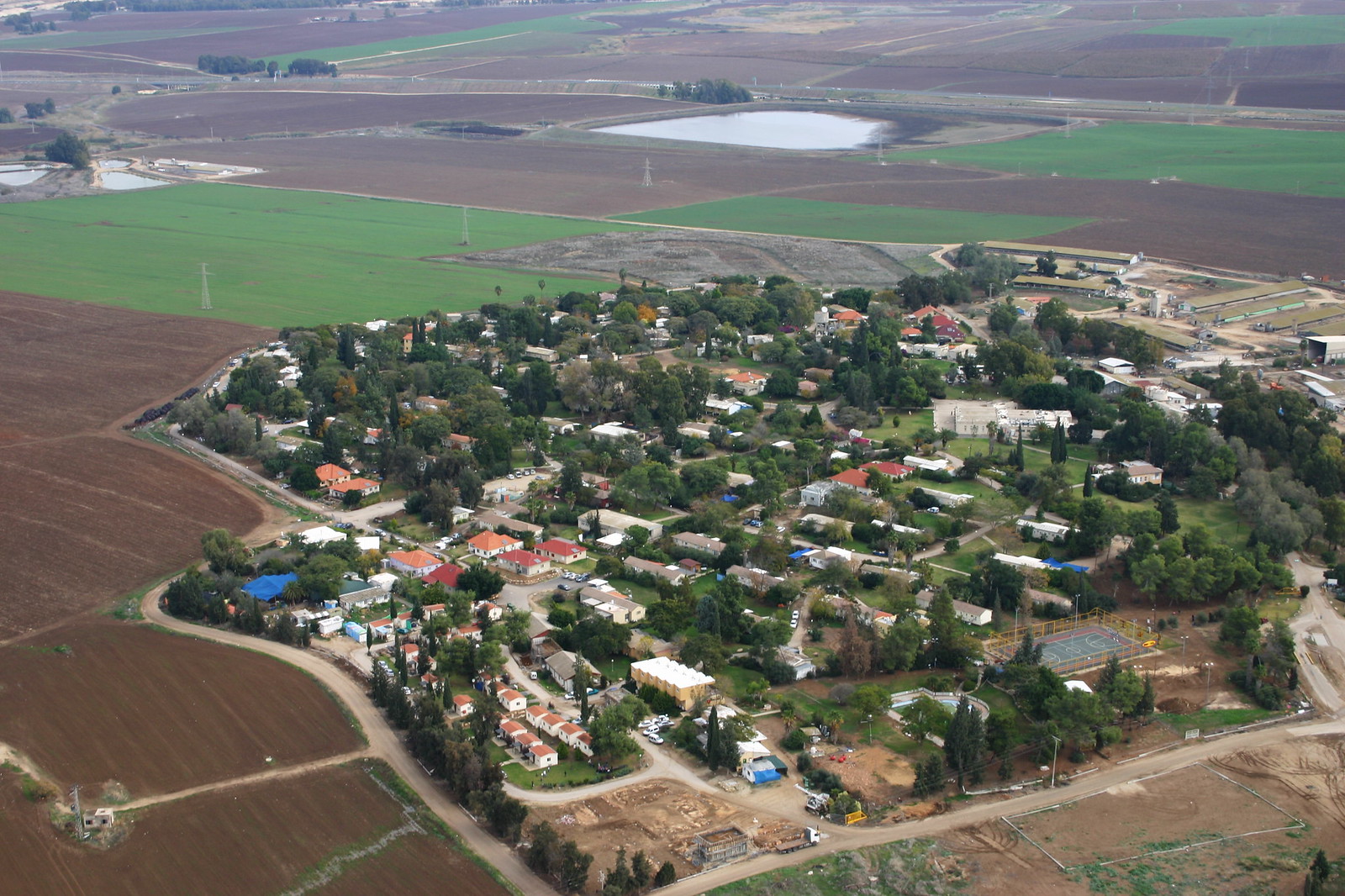This full-color aerial photograph, slightly blurry and faded, captures a small town or village surrounded by a patchwork of farmland. The image, taken on a sunny day from a plane or helicopter, showcases a community nestled amidst green grassy plots and brown fields recently tilled by farming equipment visible in the lower left-hand corner. The town center is detailed with numerous trees, various buildings, streets, and several housing units, including trailers. A tennis court is noticeable on the right-hand side, near a collection of buildings and an area of gray land situated towards the middle upper part of the image. The predominant colors of the scene are earthy browns, lush greens, and clear blues, depicting a vibrant, bustling farming community.